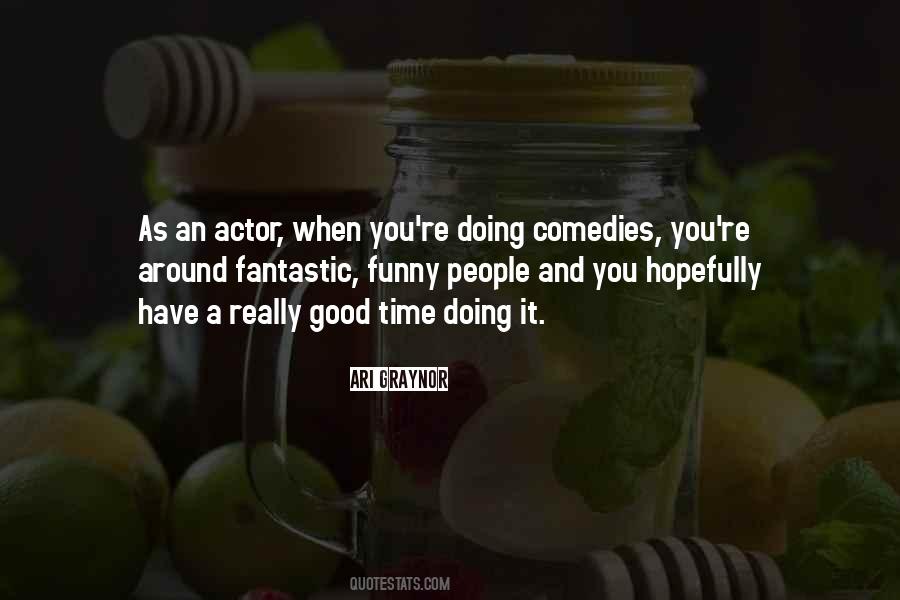The image features a centered quote in white text that reads, "As an actor, when you're doing comedies, you're around fantastic, funny people, and you hopefully have a really good time doing it." This quote is attributed to Ari Greynor, with her name highlighted in white and the text in brownish color, and below this is the source, "quote stats.com." The background of the image is somewhat dimly lit, displaying a variety of fruits including lemons and limes. There are two glass pitchers or jars prominently featured. The jar in the foreground, which has a handle and a yellow screw top, contains a mix of fruits and leaves. The jar in the background has a wooden top with a wooden-handled mixer resting on it. Overall, the background serves as a subtle yet colorful juxtaposition to the striking, centered text, lending an inviting, homemade feel to the composition.